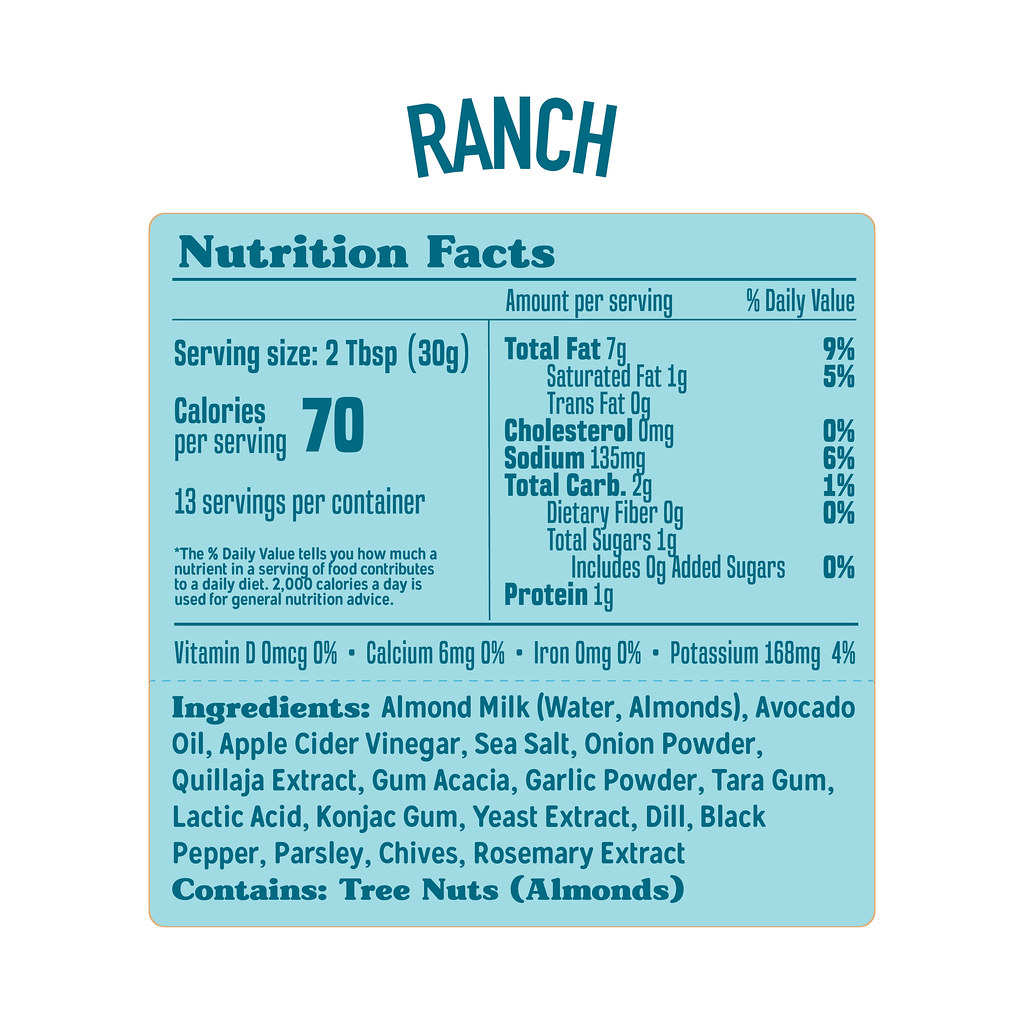The image features a detailed nutritional information label for ranch dressing. At the top, the word "Ranch" is prominently displayed in blue letters, serving as the title of the menu. Below this, a light blue box encloses the term "Nutrition Facts" written in darker blue capital and lowercase letters.

To the right of "Nutrition Facts," key details are listed:
- Serving Size: 2 teaspoons (30 grams)
- Calories per Serving: 70
- Servings per Container: 13

The nutrient amounts per serving and their corresponding daily values are clearly stated:
- Total Fat: 7 grams (9% DV)
- Cholesterol: 0 milligrams (0% DV)
- Sodium: 135 milligrams (6% DV)
- Total Carbohydrates: 1 gram (0% DV)
- Protein: 1 gram

Additionally, it mentions vitamins and minerals that are not significant in this product, such as:
- Vitamin D: 0 micrograms (0% DV)
- Calcium: 6 milligrams (1% DV)
- Iron: 0 milligrams (0% DV)
- Potassium: 168 milligrams (4% DV)

The ingredients list is comprehensive:
- Almond Milk
- Avocado Oil
- Apple Cider Vinegar
- Sea Salt
- Onion Powder
- Konjac (Coquilla) Extract
- Gum Acacia
- Garlic Powder
- Tarragon
- Lactic Acid
- Collagen
- Gum Yeast Extract
- Dill
- Black Pepper
- Parsley
- Chives
- Rosemary Extract

A final note at the bottom indicates that the product contains tree nuts, specifically almonds, and includes a warning label to that effect.